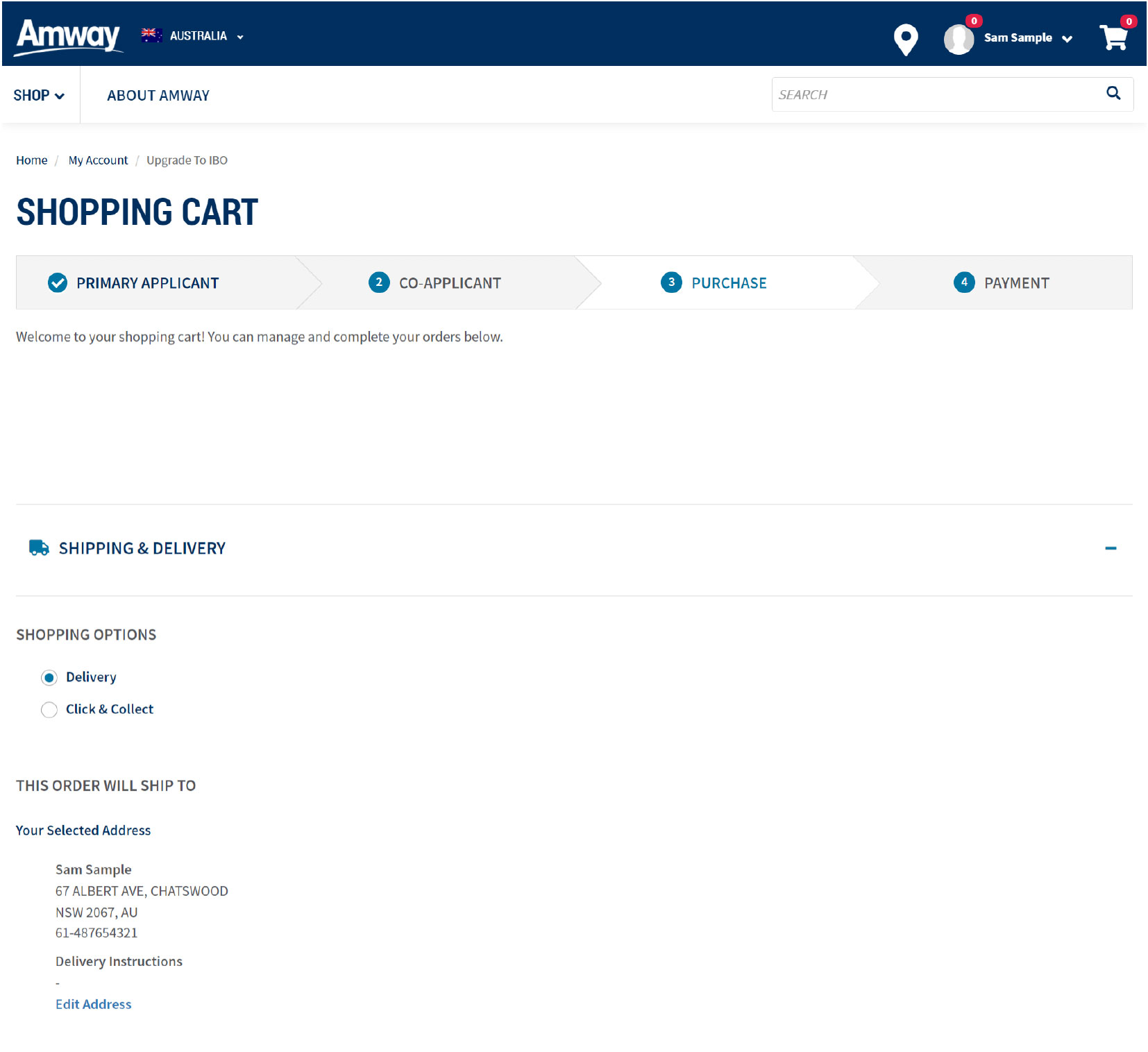**Detailed Caption:**

The image features a webpage from the company Amway, displaying a user interface prominently branded with Amway's logo and options. In the upper left-hand corner of the webpage, there is a blue header bar. On this bar, "Amway" is written in white letters with a capital 'A', accompanied by a curved line beneath the text. To the right of the logo, there is a small Australian flag followed by the word "AUSTRALIA" in all capital, white letters.

In the upper right-hand corner, there are several icons and tabs: a location finder, an avatar representing the user's account which shows the name "Sam Sample," and a shopping cart icon indicating there are currently zero items in the cart. The word "SHOPPING CART" is displayed in bold, capital blue letters.

Below the header bar, there is a horizontal navigation bar with clickable options: "Primary Applicant," "Co-Applicant," "Purchase," and "Payment." Additionally, there is a dropdown menu titled "Shipping and Delivery," offering two options: "Delivery" and "Click and Collect," with the "Delivery" option selected. 

Further down, the page states "THIS ORDER WILL SHIP TO" in capital letters, followed by the user’s selected address: "Sam Sample, 67 Albert Avenue, Chatswood, NSW 2067 AU."